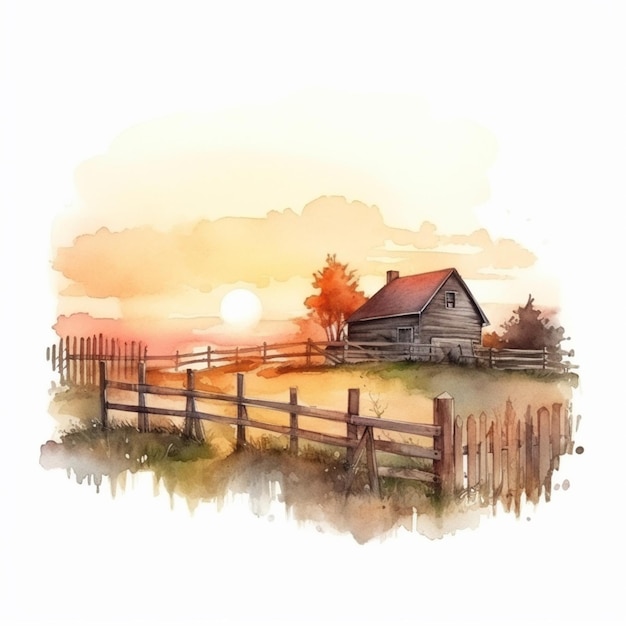In this detailed AI-generated watercolor painting, a vibrant barn scene is depicted at either sunrise or sunset, with the sun positioned on the horizon in the left distance, casting warm red and orange hues across the sky and surrounding trees. The foreground features a rustic wooden fence, with vertical posts on one side and horizontal beams on the other, enclosing a grassy yard. This lush green grass contrasts with the warm tones of the sky. The central focus is a charming wooden barn, which has one upper window and a prominent barn door on the facing wall. The barn itself has a slightly reddish tinge, while its roof exhibits a pinkish hue. A lone chimney tops the structure, adding to its quaint charm. Nestled nearby are a few trees, some of which reflect the orange and purple shades of the setting sun, enhancing the scene's picturesque quality. The softly colored clouds in the sky, painted in pink and orange, contribute to the tranquil atmosphere, while long shadows stretch across the grass, adding depth to this beautiful and serene image.